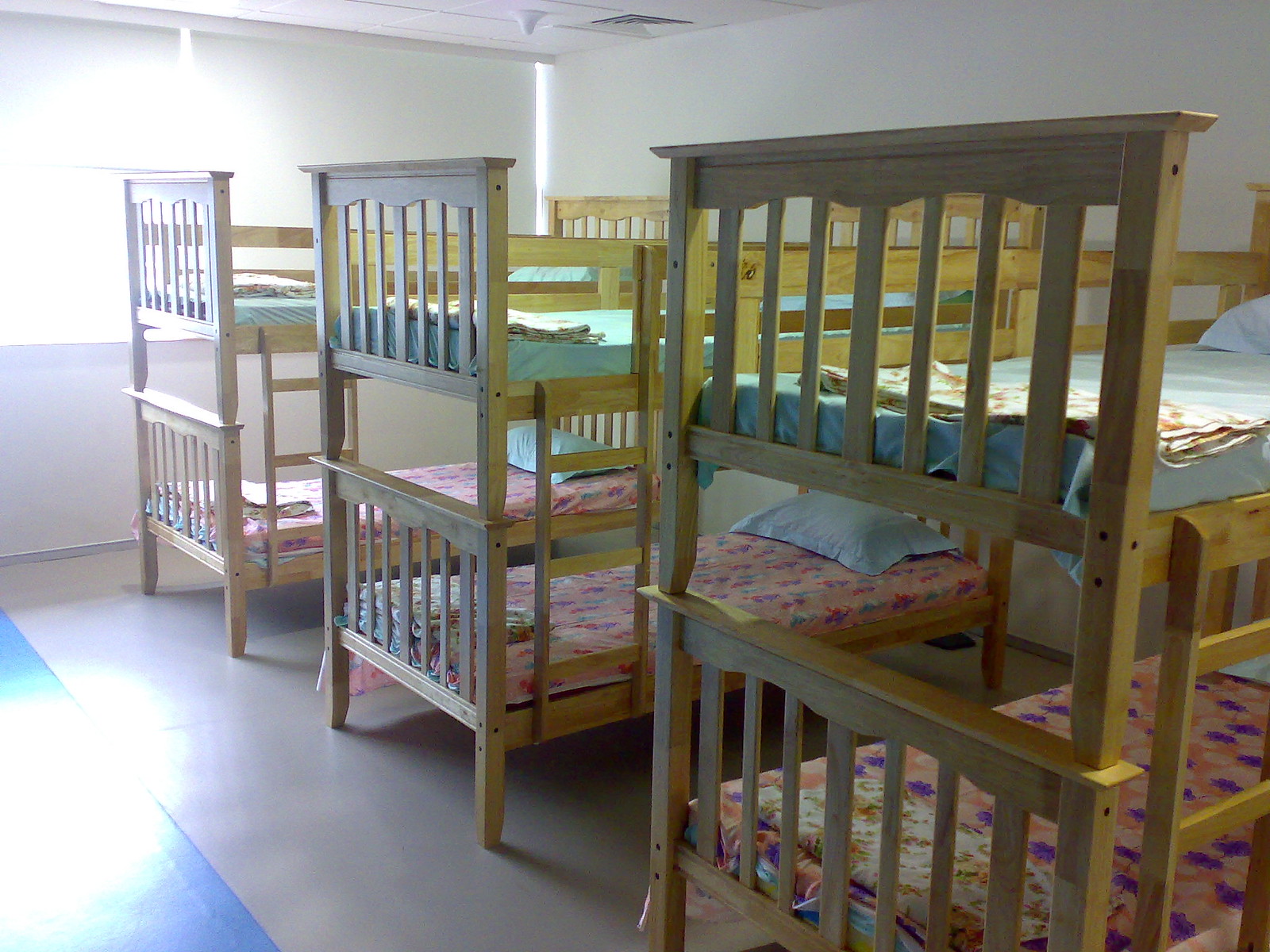The image depicts a room with pristine white walls, reminiscent of a hospital or school dormitory. The room features a solid linoleum floor, and in the far left corner, sunlight filters in through a window, casting a bright glare onto a blue rug. Dominating the space are three sets of wooden bunk beds, crafted from light pine wood, arranged along the far right wall with just enough space between them for a person to walk. Each bunk bed consists of a top and bottom bed, both equipped with neatly tied fitted sheets. The top bunks are adorned with solid light blue fitted sheets, blue pillows, and folded blankets at the foot of the bed. The bottom bunks contrast with pink sheets, decorated with a purple floral pattern, and matching blue pillows and folded blankets. The overall neatly organized setup and the functional design suggest a shareable, utilitarian bedroom designed for multiple occupants.